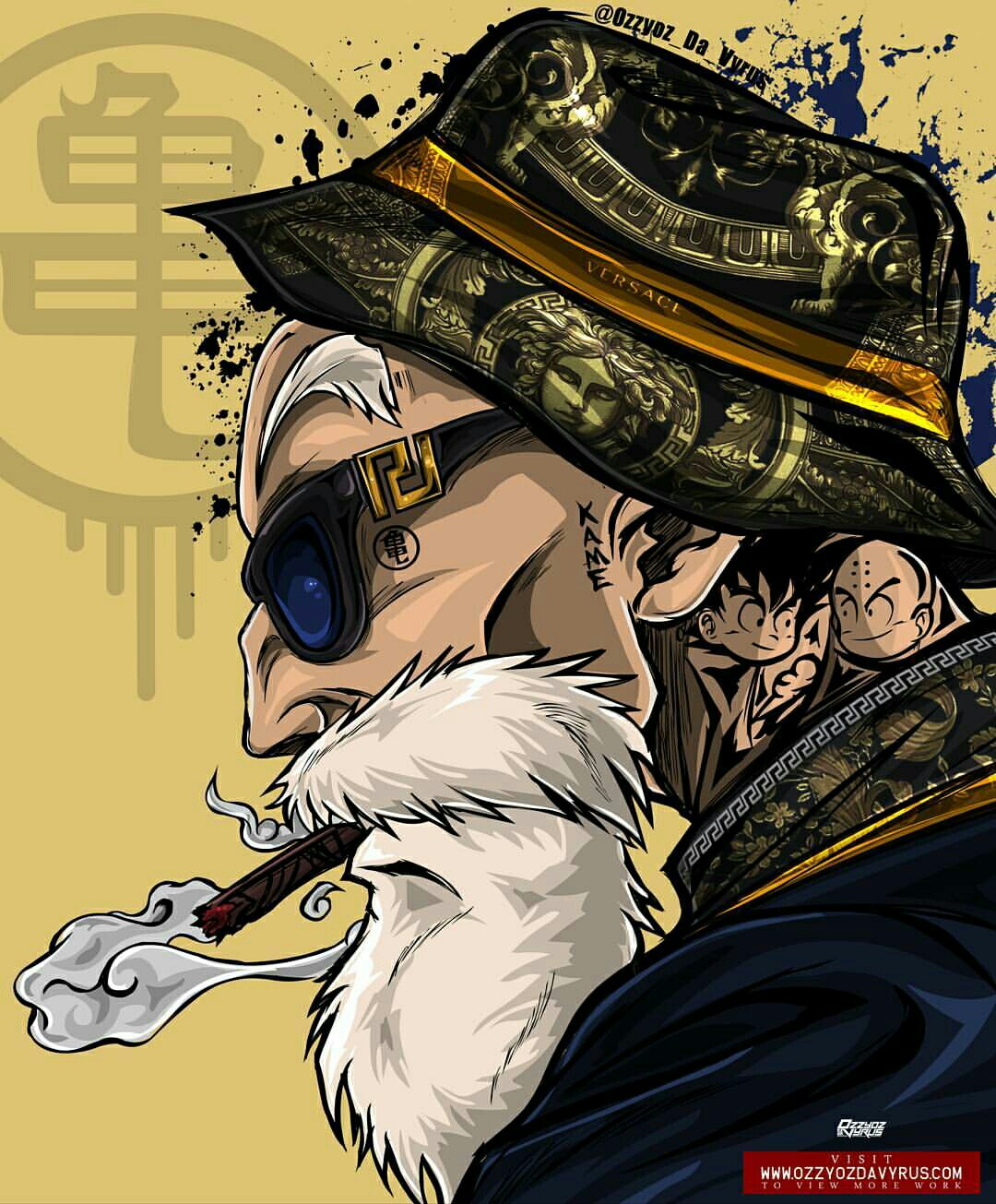In this colorful and stylized cartoon drawing, an older man, facing left, is depicted with intricate detail. He sports a distinctive black and light gold Versace hat, adorned with a gold band bearing the brand name. His bushy white eyebrows contrast with his black and blue sunglasses that feature a small gold logo. His face, shaded in tan, is complemented by a large white beard from which a smoldering cigar protrudes, releasing a trail of smoke. On the side of his face, near his ear, the initials "K-A-M-E" are engraved. His neck showcases a tattoo of two grimacing children, adding an element of intrigue. He dons a dark blue jacket with a highly stylized and ornate collar, enhancing his eccentric appearance. The background is awash in a vibrant yellow, accentuated by a circular symbol with lines and a red logo with text at the bottom right. The bottom of the image contains the small and scarcely legible text “VisiteeAussieDaverRuss.com,” adding to the enigmatic allure of this detailed composition.